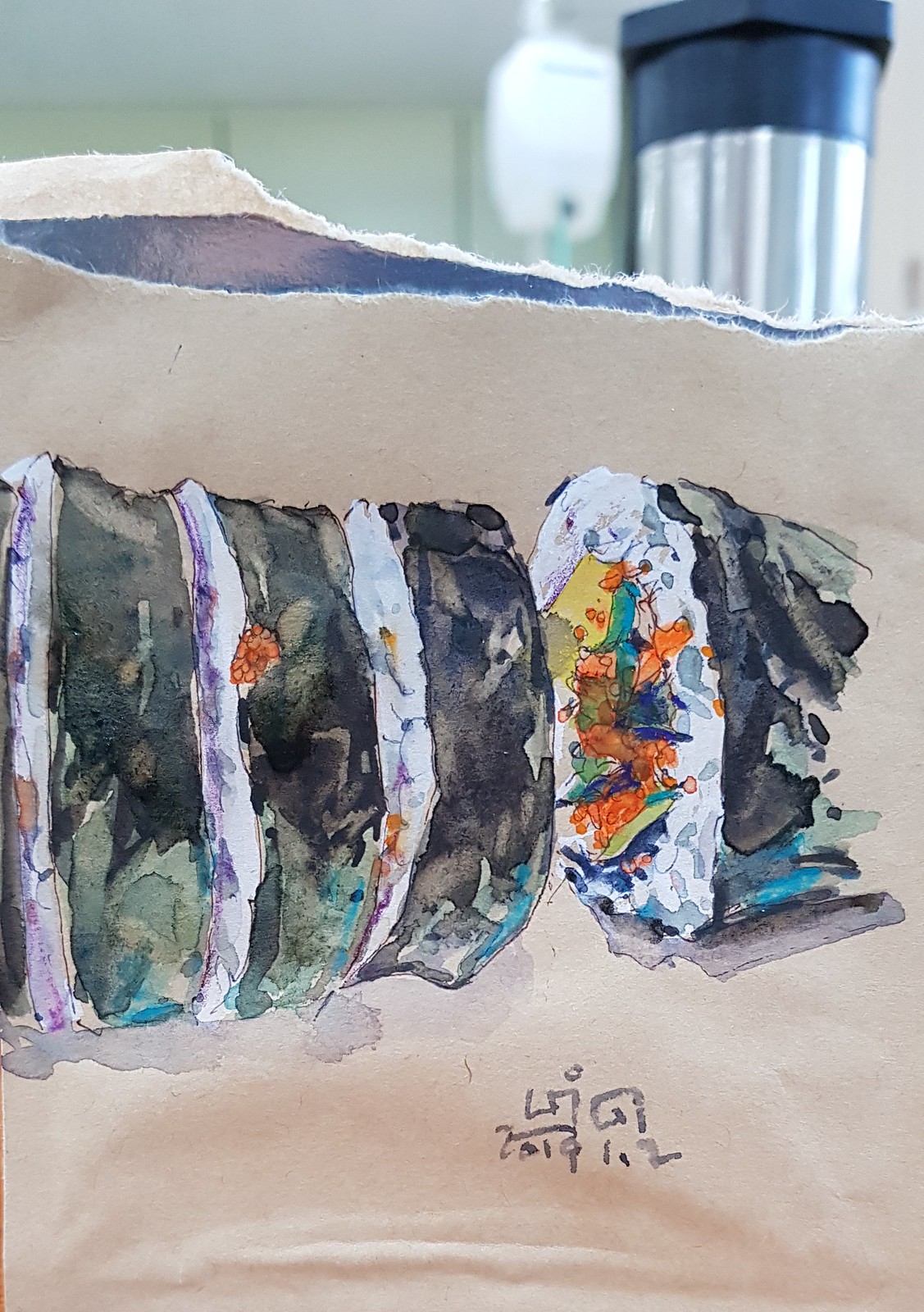This color photograph depicts a detailed watercolor painting of sushi on a piece of thick, cream-colored, textured paper. The paper is slightly torn at the top, revealing a bluish edge underneath, suggesting it is overlaid on another, similarly torn piece of paper painted blue. The artist’s signature, written in an Asian script, and the date "2019-1-2" are visible at the bottom of the painting.

The sushi itself is intricately painted, capturing the various components and colors evocatively. It features a greenish-black wrapper with white sections that represent rice, shaded in gray. Inside the rice, the filling includes vibrant orange fish roe and additional elements painted in shades of blue, green, teal, and yellow, creating a colorful mosaic. The depiction includes thoughtful shading, with some sections highlighted in purple and lavender, adding depth and realism to the piece. In the background, at the top of the image, a greenish-grey tiled wall is visible, along with a blue-topped object on the right that has a metallic silver base with vertical lines and an unlit white light in its center.